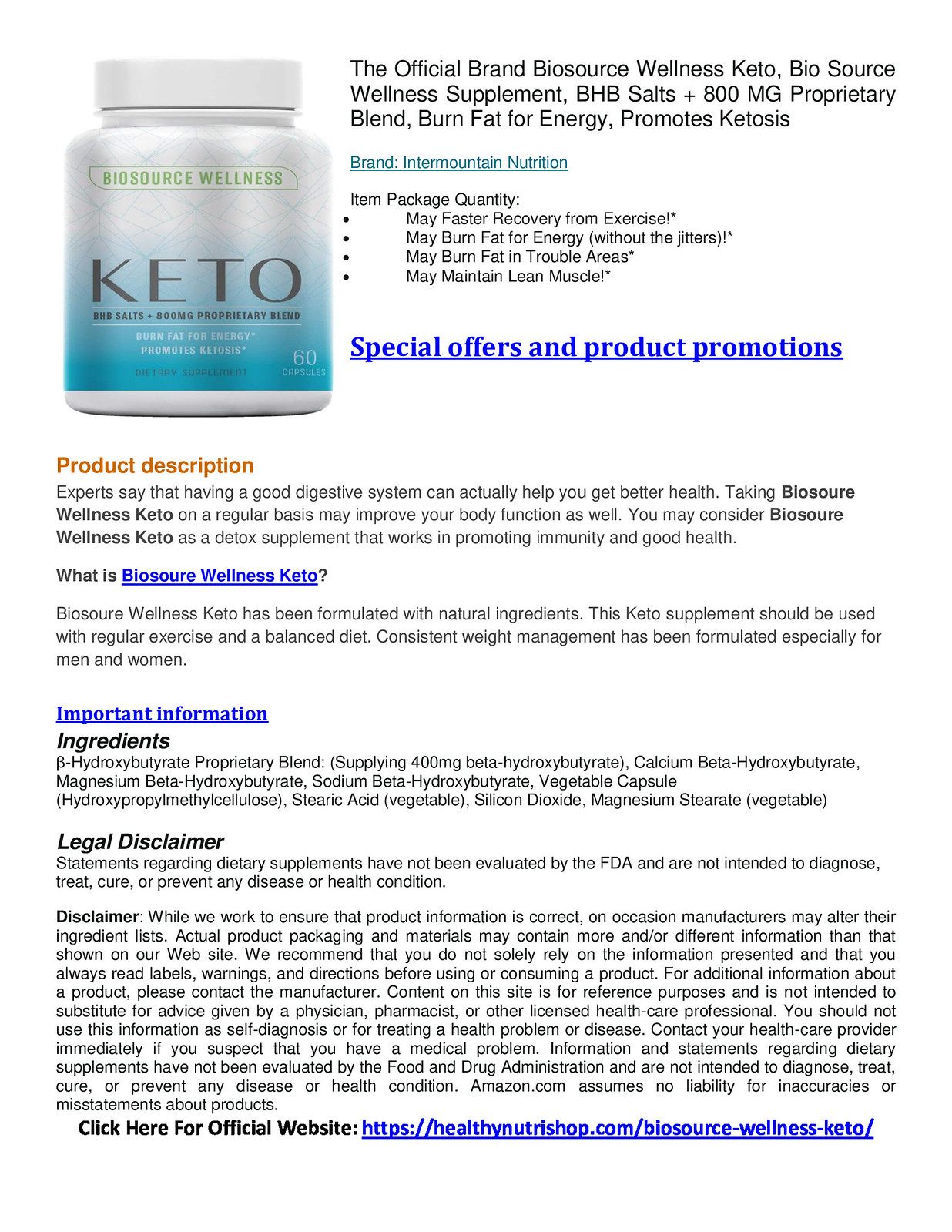**Product Description Screenshot for Biosource Wellness Keto Supplement**

In the upper left corner of the image, there is a small plastic bottle with a round cap. The bottle features a white label that transitions to a light blue color towards the bottom. Prominently displayed in black capital letters on the lower half of the label is the word "Keto." Above this, within a green oval outlined in blue, it reads "Biosource Wellness."

To the right of the bottle and occupying the majority of the image below it is extensive printed information. At the very top left, it states, "Official Brand: Biosource Wellness Keto." It is followed by the product name, "Biosource Wellness Supplement," along with key details such as "BHB Salts plus 800 mg," "Proprietary Blend," "Burn Fat for Energy," and "Promotes Ketosis."

Below this header is a detailed product description, outlining the benefits and features of the supplement. Further down, the section contains important information, including a comprehensive legal disclaimer.

At the bottom of the image, there is a call-to-action or link labeled "Click Here for Official Website," which directs to: [https://healthynutritionshop.com](https://healthynutritionshop.com)